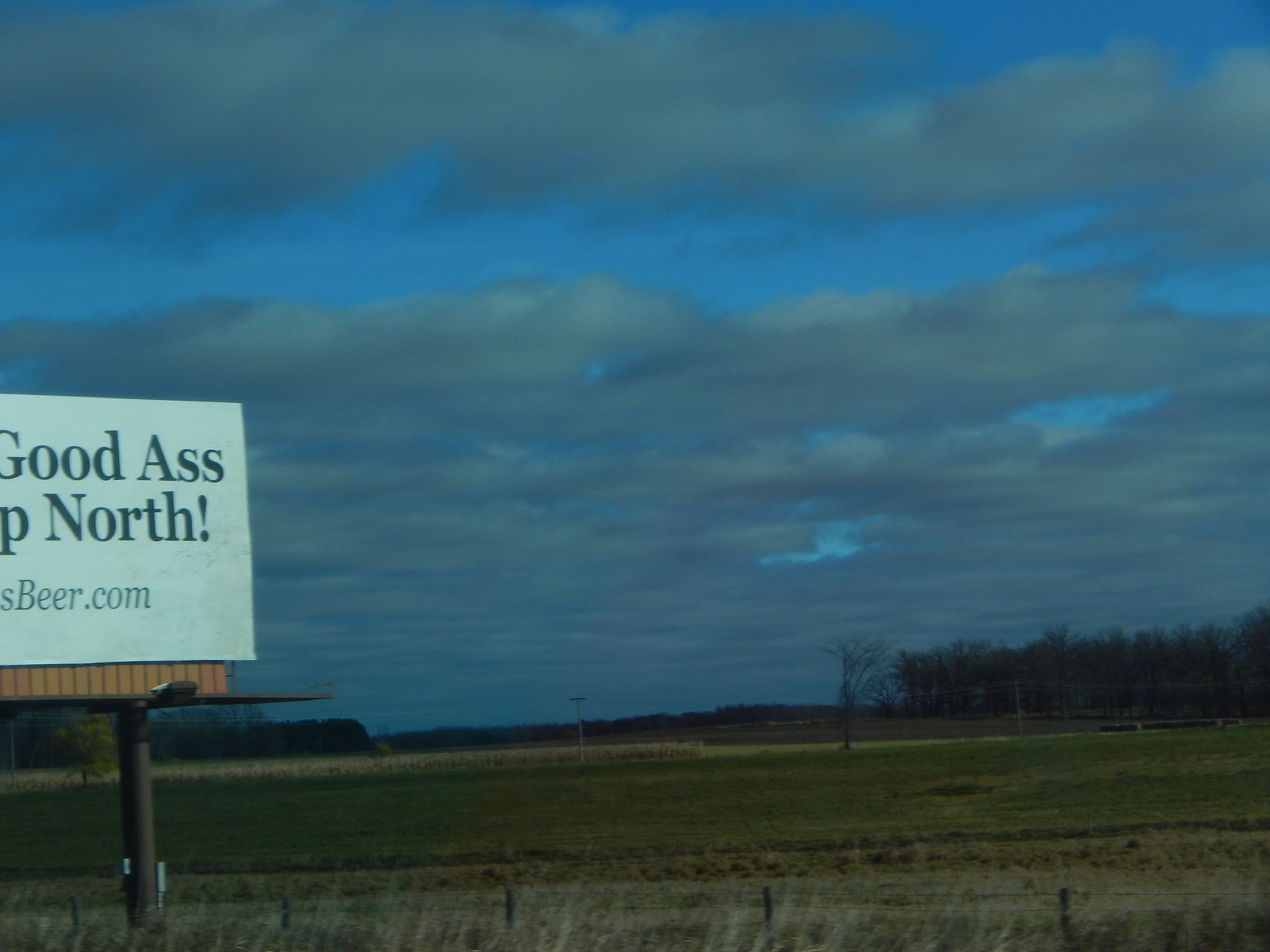The image captures an expansive outdoor scene dominated by a sky that spans the majority of the frame. The sky features a palette of light blue and light gray tones, interspersed with an array of gray clouds. To the left of the image stands a partially visible white board, prominently displaying the text "GoodASS! Bear.com." Behind this board, a lush field of green grass stretches out, adding a vibrant contrast to the muted hues of the sky. The overall composition highlights the vastness of the sky while providing intriguing details in the foreground with the board and the verdant field.